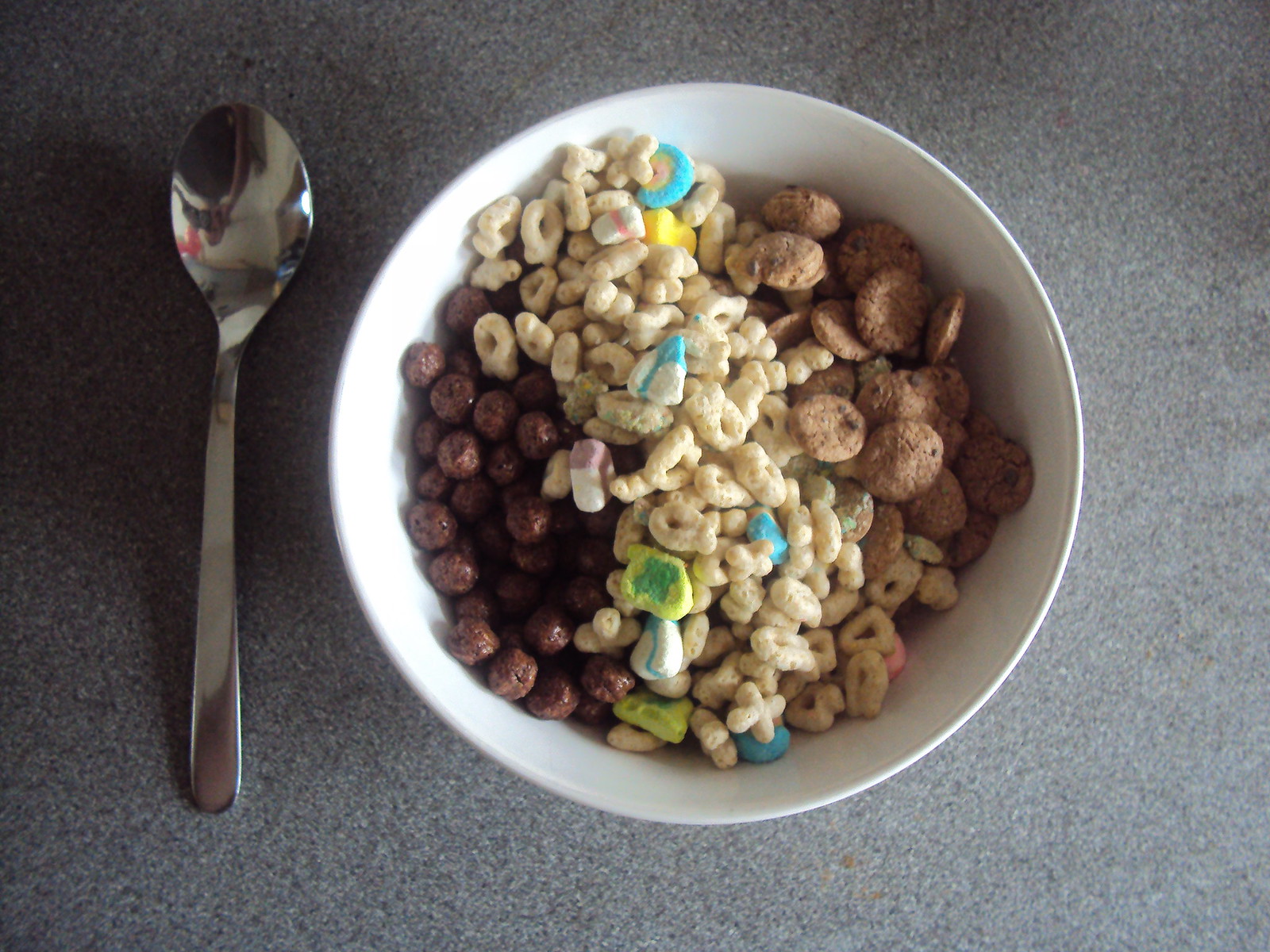The image features a top-down view of a full white cereal bowl placed on a gray speckled laminate countertop. Positioned centrally, the bowl contains three distinct types of cereal arranged in separate columns. On the left side, there are dark brown, round discs resembling Cocoa Puffs. The middle section is filled with oat-shaped cereal pieces interspersed with colorful candies, including blue and lime green pieces, likely resembling Lucky Charms. On the right side, lighter brown puffed circles, possibly similar to Cheerios or another type of crispy cereal, can be seen. To the left of the bowl is a reflective silver spoon, pointing upwards towards the ceiling.